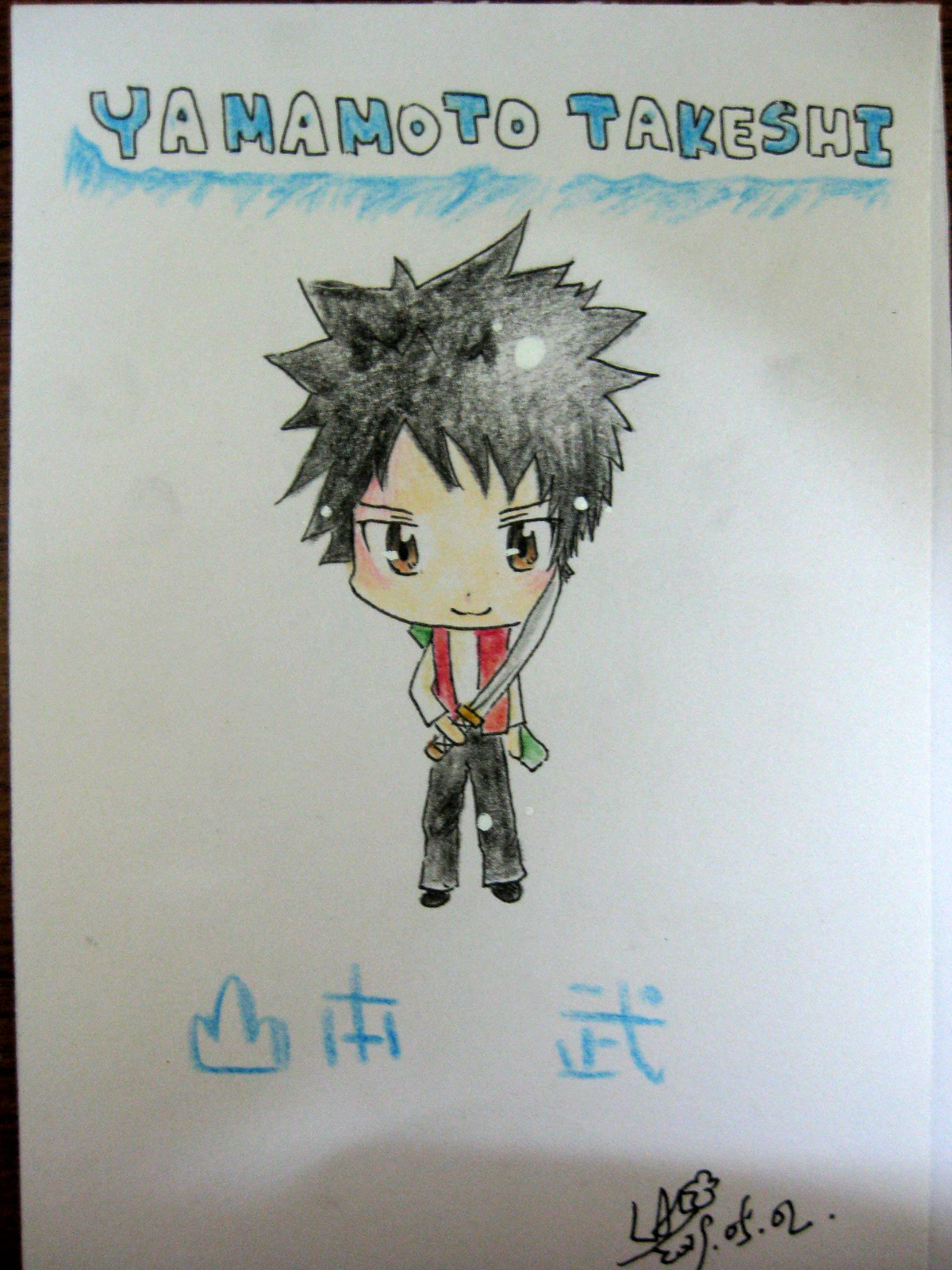This drawing showcases an anime character named Yaramoto Takashi. The image captures Takashi with a disproportionately large head, adorned with spiky black hair and large brown eyes. He is depicted smiling and holding a sword in one hand, while a green sheath can be seen on his back. Takashi is dressed in a recognizable outfit consisting of a white shirt, a red vest, black pants, and black shoes. The portrait is vividly colored, with a particular emphasis on the character's attire and accessories.

At the top of the image, his name, Yaramoto Takashi, is prominently displayed with alternating blue and white letters, giving it a shimmering appearance. The white background of the drawing keeps the focus on the character. Below the figure, there are Japanese symbols and an autograph signed in black ink, adding to the authenticity and detail of the piece. Despite being described as a child's drawing, it bursts with vibrant colors and personality, making it a charming representation of an anime character on a simple, white canvas.